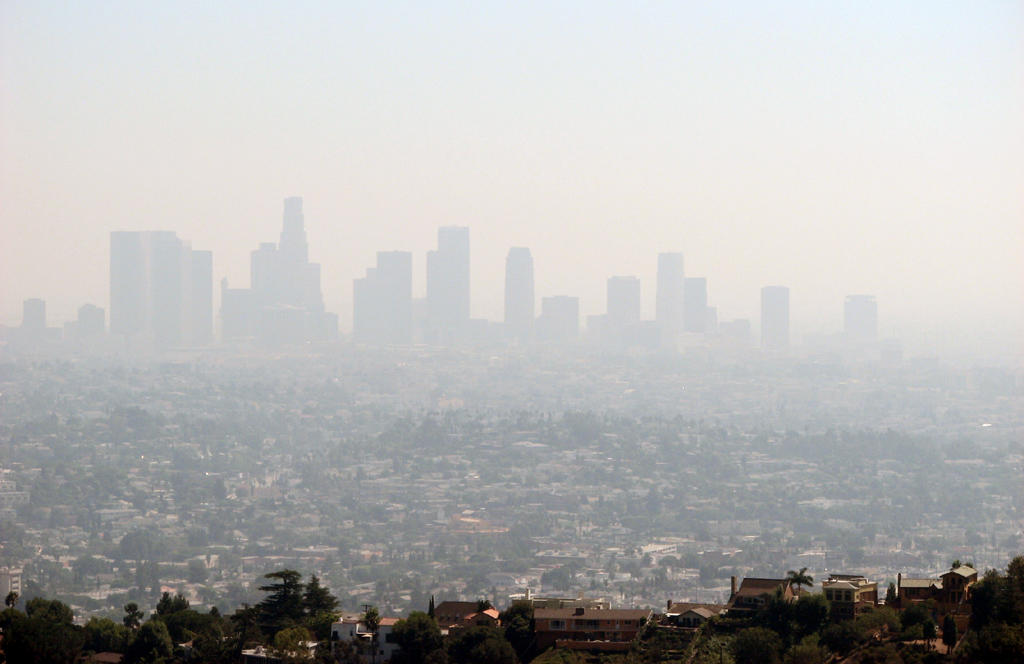The image captures a hazy daytime view of Los Angeles from a large, tree-covered hill adorned with affluent residential housing. In the foreground, the hillside is dotted with rich-looking homes, surrounded by lush foliage and palm trees, indicating the warm climate. The scenery transitions from these affluent neighborhoods to densely packed suburbs filled with smaller buildings interspersed with trees. Dominating the distant background, the Los Angeles downtown skyline juts into the sky with numerous tall skyscrapers, particularly clustered towards the left side. The entire cityscape is enveloped in a thick layer of smog, giving it a smoky, almost fog-like appearance, which softens the visibility of structures and creates a hazy ambiance across the sprawling urban landscape.